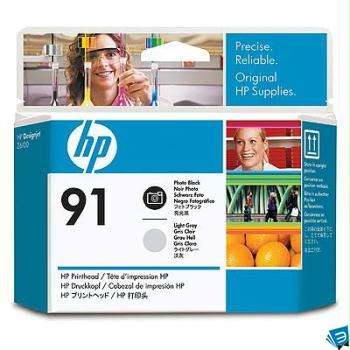This detailed description combines elements from all three captions:

The image depicts a blue rectangular box for HP 91 printer ink, featuring angled sides. Dominating the front is a white circle with the lowercase letters "hp" and below it, a white rectangle displaying the number "91" in black. To the right, there's a symbol of a camera. Above the main section, a banner features a woman with shoulder-length, frizzy curly hair, wearing lab glasses. She is holding a test tube in front of her, with another test tube positioned to the left side of her face. The setting appears to be a laboratory with a visible hanging light on the right. Adjacent to her image is a blue rectangle with white text reading, "Precise, Reliable, Original HP Supplies." Additional details on the box include the words "HP 91" indicating photo black and light gray ink, alongside multilingual text describing its reliability. The cohesive blend of blue and white colors with accents of other hues completes the packaging design.